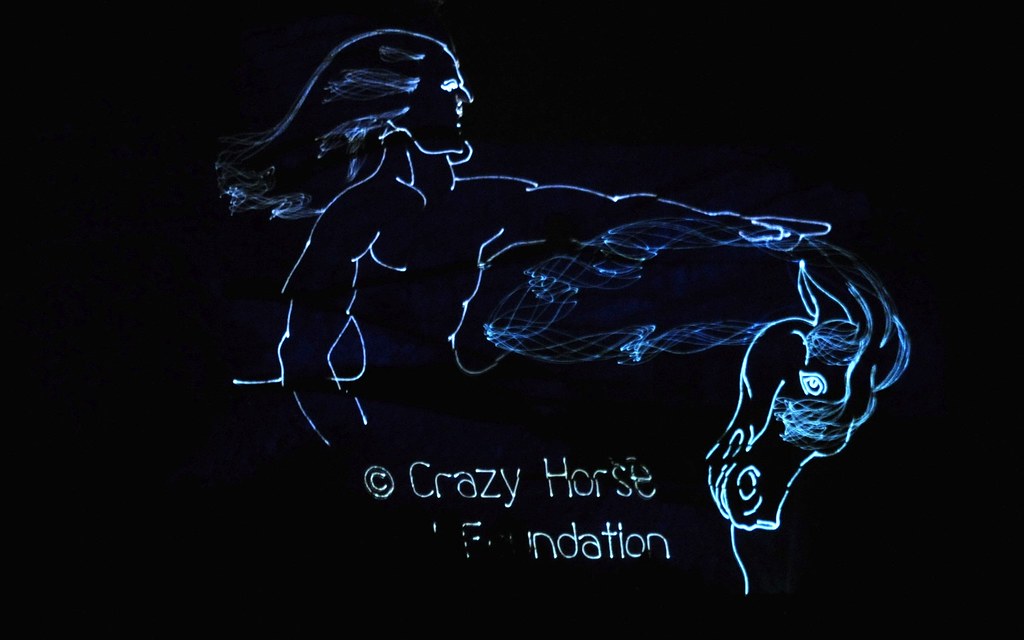The image features a detailed illustration on a deep black background, likely rendered with chalk or metallic gel ink in a glowing blue-white hue. The central figure is a muscular, long-haired man depicted in a minimalist line drawing style, with his torso exposed and his left arm outstretched over the head of a horse, which is positioned on the right side of the image with its head lowered. The man's right arm appears relaxed by his side. The illustration is simplistic yet dynamic, capturing the flowing motion of both the man's hair and the horse's mane. Below this evocative scene, the text "Crazy Horse Foundation" is inscribed in a matching graphic style.